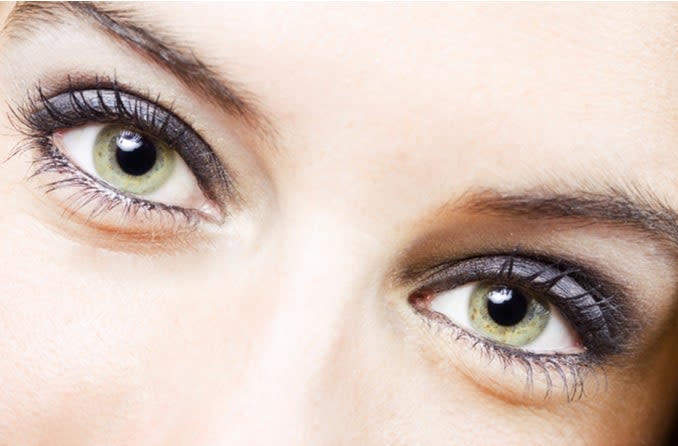This close-up photograph captures the intense and arresting gaze of a Caucasian woman with light-colored skin. Her eyes are prominently green with flecks of brown and gold, framed by thin brown eyebrows and dilated black pupils. Her lashes are heavily coated in mascara, giving them a long, voluminous look, while her eyelids are adorned with a smoky dark gray eyeshadow that extends to a hint of silver on her lower lids, accentuated further by gray eyeliner. Her skin appears smooth and clear, with no visible blemishes, and her serious expression is magnified by the dramatic makeup. The composition has her head tilted slightly, positioning one eye in the upper left and the other closer to the lower right, drawing attention to the intricate details of her eye makeup and the clear, sharp features of her face.